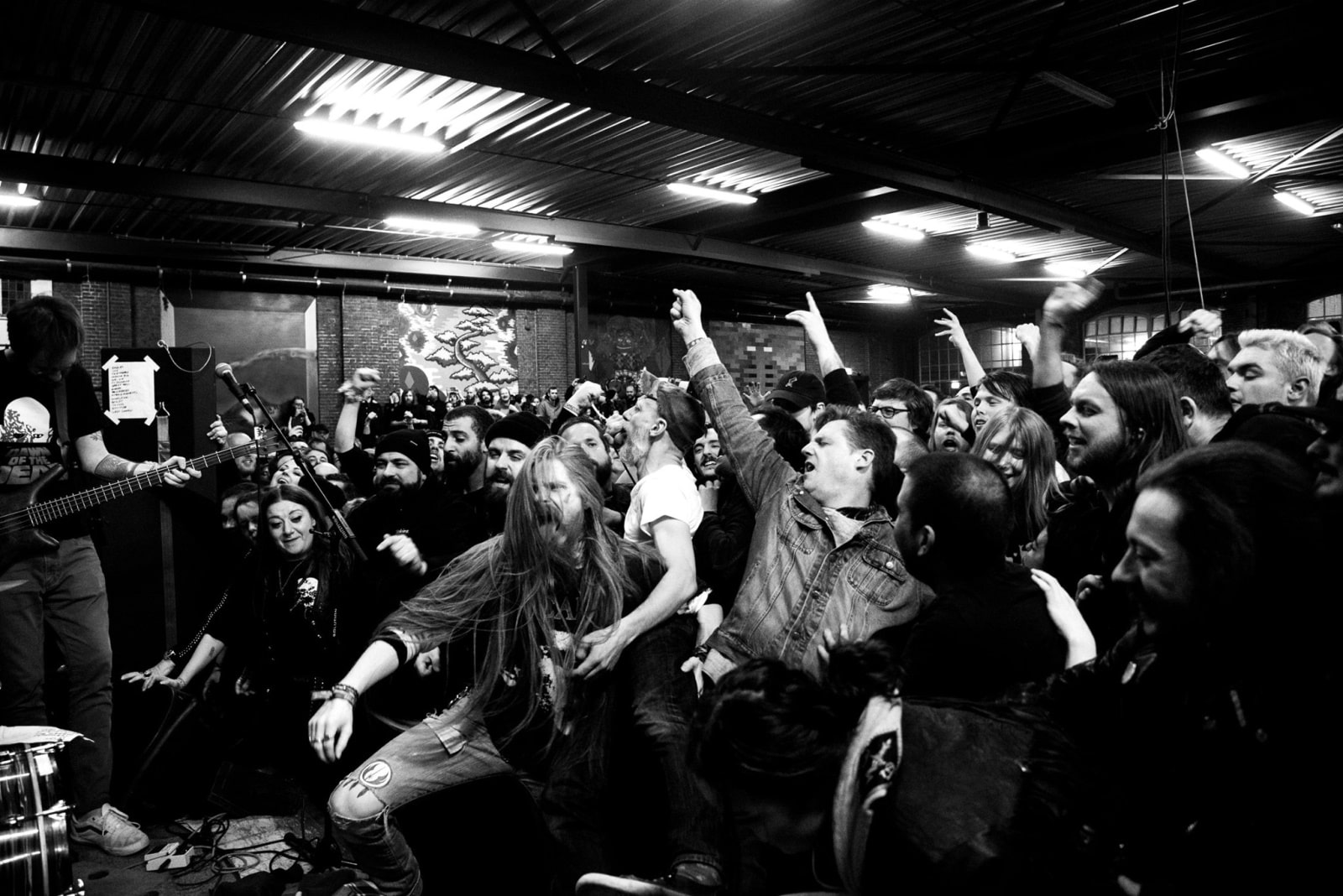This black and white landscape photograph captures the electrifying atmosphere of a small, packed rock venue during a live performance. On the left-hand side, a man with a bald head, dressed in a black T-shirt, is partially visible, focused intently on his electric guitar, cut off at the pickups. In the foreground, a stool rests, and a drum is visible on the stage, adding context to the setting. 

The crowd, tightly packed and energized, has their hands in the air, with some individuals nearly climbing onto the stage. A standout figure, a man with extremely long hair and ripped jeans, is seen with one knee practically on the stage, embodying the intensity of the moment. Next to him, a young lady reaches out her hand towards the stage. Other attendees are pointing, singing, and headbanging, fully immersed in the experience. The ceiling above, lit with metal slats, completes the intimate yet intense atmosphere of this indoor heavy metal club.